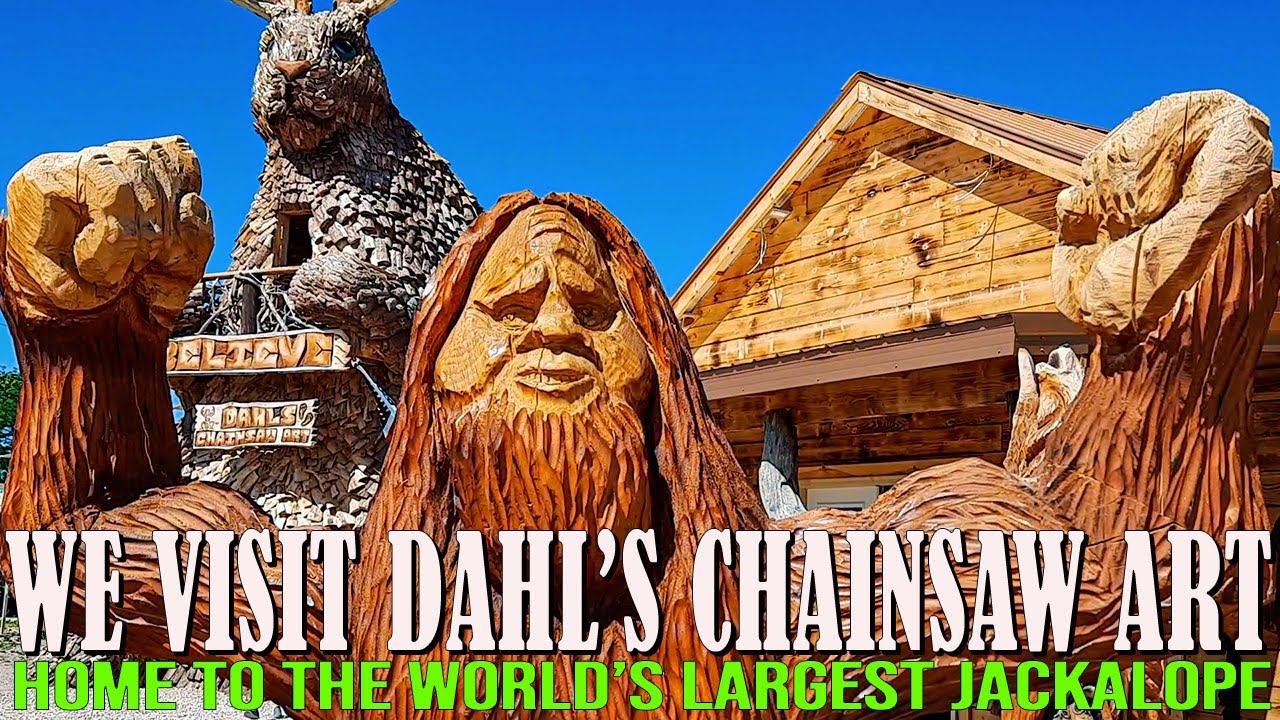In front of a rustic wooden cabin, there's a detailed wooden carving of a Yeti, or Sasquatch, characterized by exaggerated facial features, large hands, pronounced muscles, and a scraggly beard, all rendered with meticulous chainsaw detailing to depict a hairy texture. Situated behind the Yeti to the left is an extremely tall rabbit with horns - a giant wooden jackalope. This jackalope holds a sign with a window cut-out in its chest and features stairs and a door for entry. The scene is set against a clear blue sky, unmarred by clouds, with a piece of a tree visible on the left. Overlaying the top section of the Yeti is a sign in white font reading, "We Visit Dawg's Chainsaw Art," with a green-font subtext proclaiming, "Home to the World's Largest Jackalope."